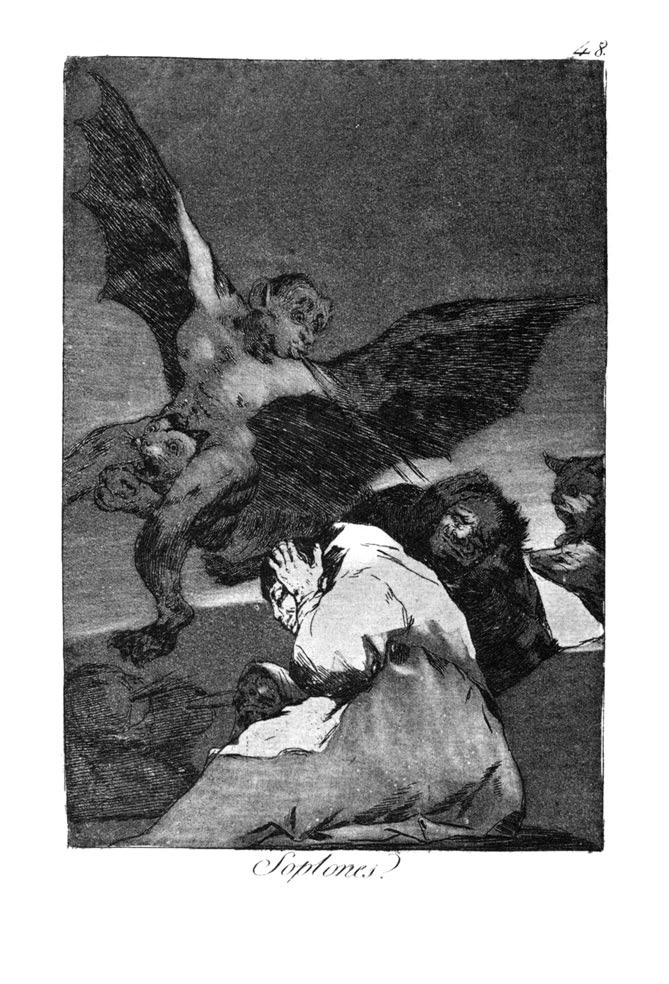In this striking monochrome artwork, a distressed figure, potentially a woman dressed in a grey dress and white top, sits on the ground with hands pressed to ears in apparent fear. Above the figure's right shoulder hovers a menacing dark creature, possibly a demon or beast. Further up, dominating the top left corner, is a fierce bat-winged demon, its face twisted in anger as it appears to spit something at the dark entity closer to the ground. To the side, another dark figure, resembling a dog, seems to bark loudly at the cowering figure. The grey sky and overall dark background add to the ominous atmosphere, with the only text, "SOPLONES," located at the bottom center. The detailed folds of the figure's garment in bright white and grey contrast starkly with the surrounding darkness, enhancing the overall tension and drama of the scene.